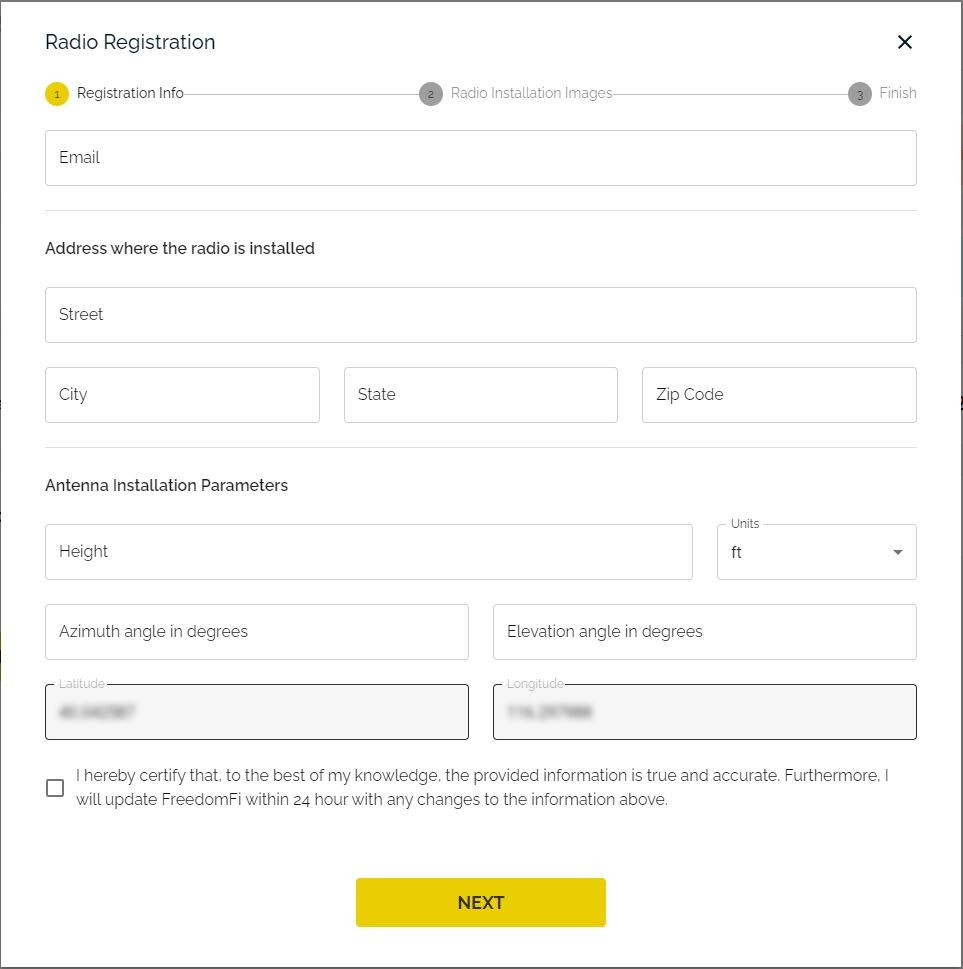This image showcases the first step of the "Radio Registration" process on a webpage. The screen prompts the user to enter several technical details, including an email address, the specific location where the radio will be installed, and various antenna installation parameters such as height, azimuth angle, and elevation angle. Additionally, it requires the latitude and longitude coordinates of the installation site. There is a certification statement at the bottom, confirming that the entered information is true and accurate to the best of the user's knowledge, and that any changes will be reported to FreedomPHY within 24 hours. A checkbox next to the certification statement must be selected before proceeding. The "Next" button, colored in yellow, allows users to move to the subsequent steps: "Radio Installation," "Images," and "Finish." The background is primarily white with black text, and occasional yellow elements highlight key actions. The overall design implies a registration process that may be linked to a satellite service or a regulatory body, given the technical nature of the required information.